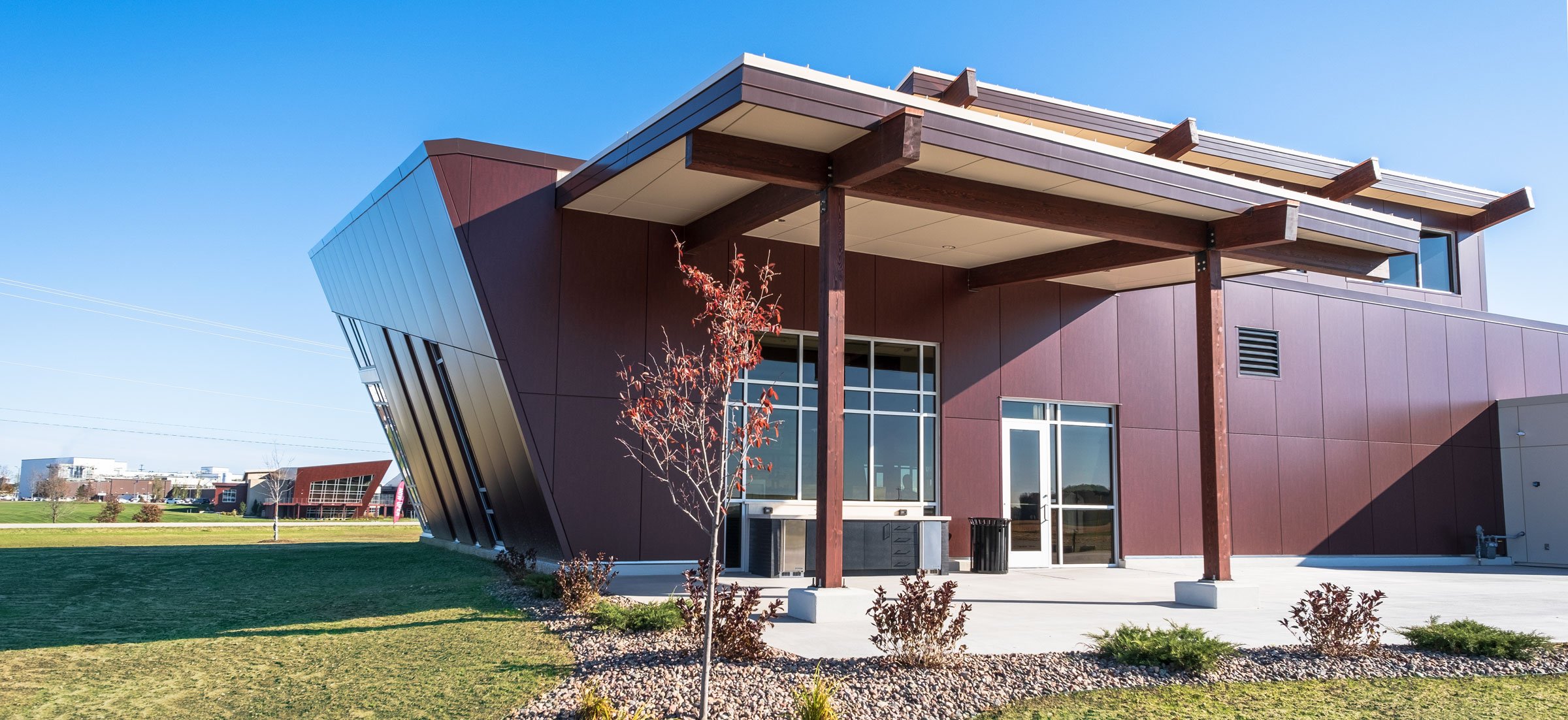The photograph captures a sleek, modern building under a big, clear blue sky, featuring maroon-colored siding. The facade is dominated by a tall glass window on the left, which may have an air conditioning unit in front of it, and a glass door with a white-trimmed panel in the center. The building could be either a contemporary home or an office-type structure. Supporting an awning, purplish stanchions contribute to its modern appeal. A concrete patio or porch area surrounds the base, equipped with what appears to be an outdoor work area with cabinets and drawers, and a trash can sits conveniently by the door. The left side of the building exhibits an intriguing slant, and a beam-supported roof, possibly tiled, adds to its architectural uniqueness. An air vent is noticeable through the siding. The building is set against a grassy expanse with small shrubs and a newly planted tree, hinting at its newness and meticulous landscaping. Far in the background, a second similar modern structure is visible, suggesting a planned community or university campus.